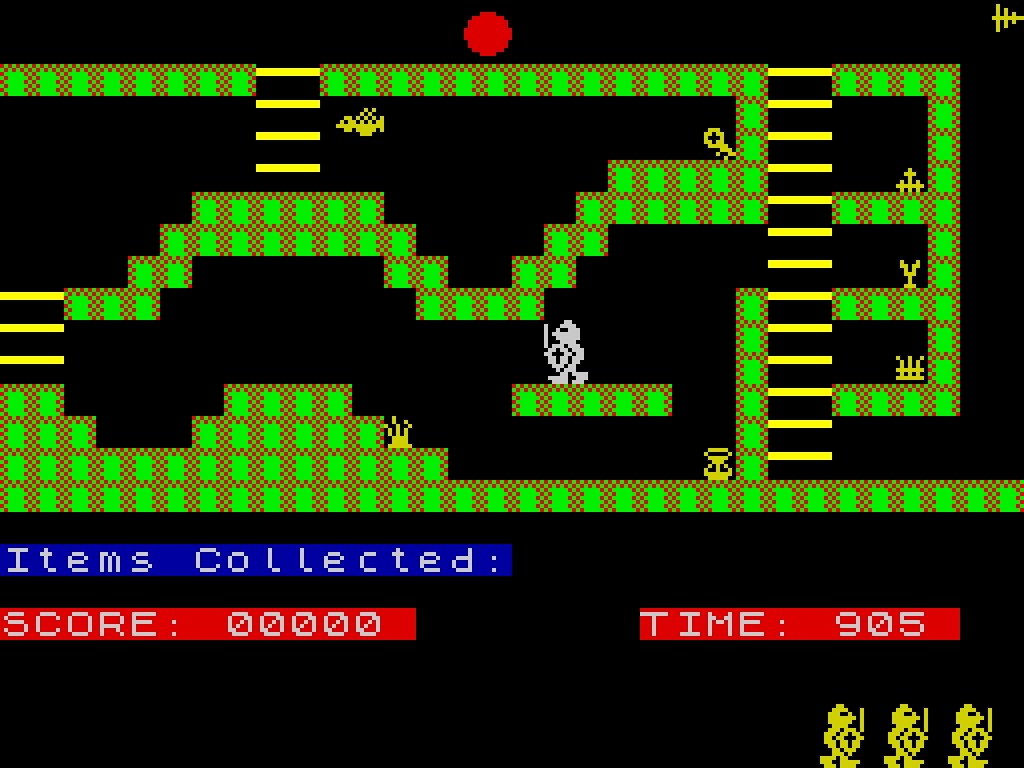In this video game screenshot set against a stark black background, a vivid, action-packed scene unfolds. Dominating the top center is a conspicuous red spot. Below it, intricate green structures stretch across the screen, punctuated with red-and-green checkered squares forming a mesmerizing pattern.

The environment is multi-leveled with yellow steps providing a pathway downward to subsequent levels. Tiny, agile birds, characterized by their yellow bodies and black-and-yellow checkered wings, flit about the scene.

In one corner, a small key gleams, hinting at an essential quest item. Central to the action is a valiant knight clad in white armor, brandishing a shield marked with a bold black cross and a ready sword, poised for battle. He navigates through various perils, with yellow characters scattered across the bottom of the frame, adding to the chaos.

Two informational boxes are prominently displayed: a blue one announcing "Items collected" in white text, and a red one displaying "Score: 0" and "Time: 905" also in white. The bottom of the screen features three small yellow figures, perhaps lives or additional characters, contributing further to the game's intricate design.